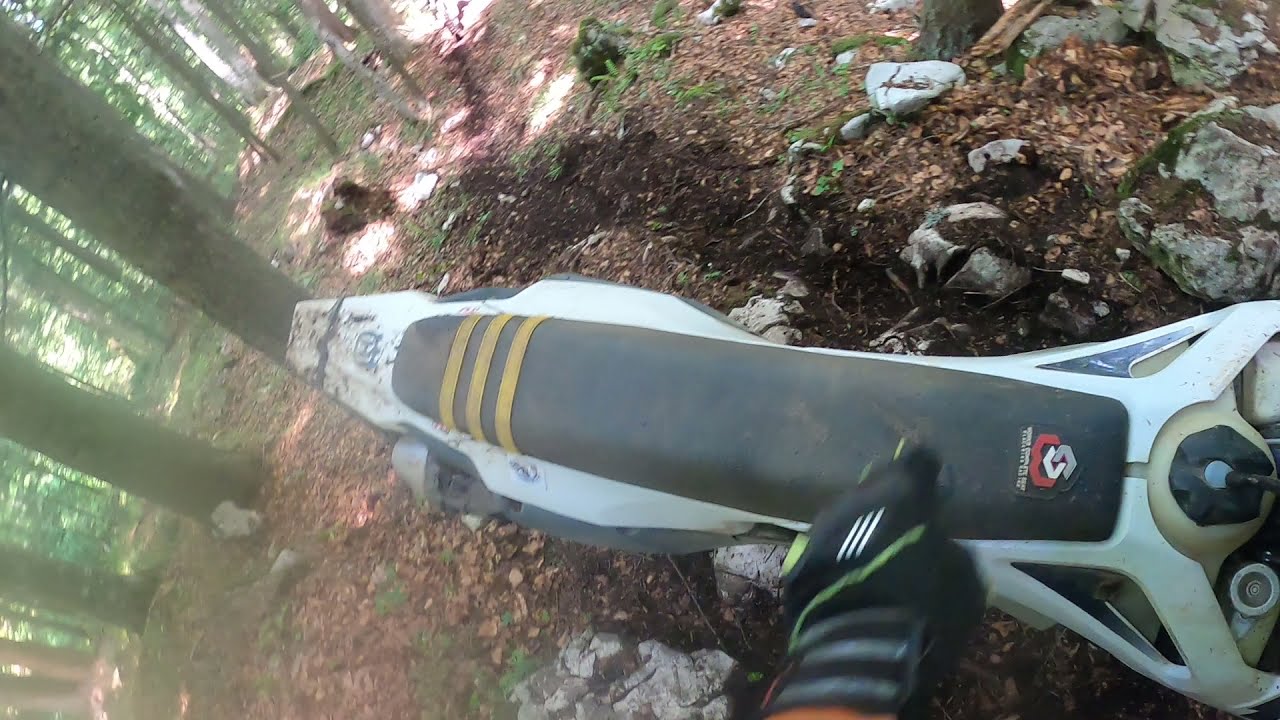In this point-of-view shot, a dirt biker is looking down at his dirt bike positioned in the center of the image. The bike features a black seat adorned with yellow stripes and a red, gray, and white interlocking logo. The body of the bike is primarily white with black trim, and the biker's black gloved hand with yellow trim is pointing at the seat. The ground beneath is covered in dark, muddy forest dirt interspersed with light gray, moss-covered rocks. On the left side of the image, the bases of several large trees can be seen, with additional trees in the distance displaying light green leaves. Sunlight filters through the tree branches on the left, casting a soft glow over the scene. The perspective suggests the biker is either standing beside or preparing to mount the bike, emphasizing the rugged, natural environment that surrounds them.